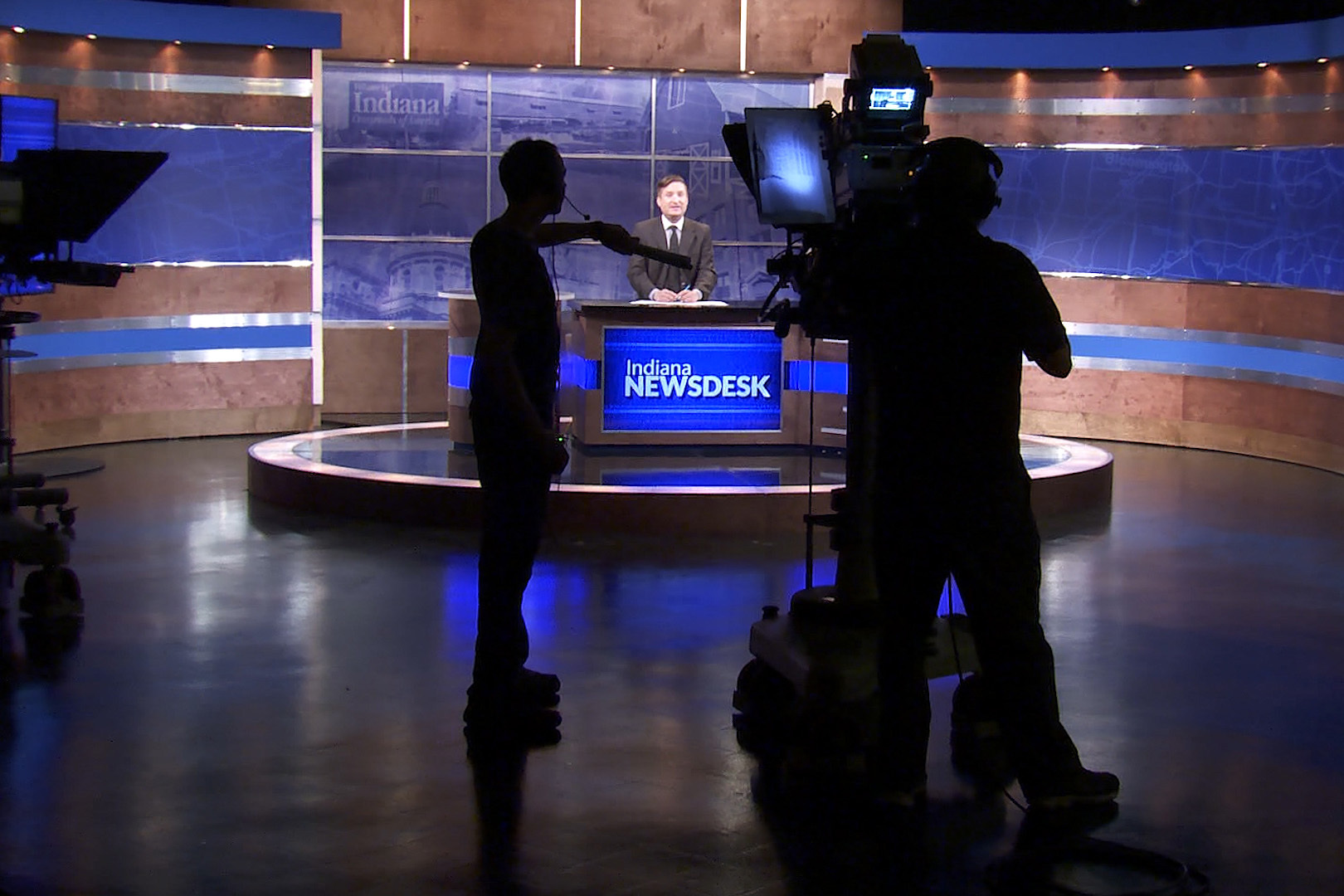The image captures a color photograph of a live television broadcast from an Indiana news studio. The shot is taken from behind two silhouetted figures: one appears to be a director or showrunner, wearing a microphone headset and gesturing with his hand on the left, while the other operates a large camera on wheels, positioned to the right. Both men are working in front of a sleek, smooth black floor. Centrally, a man in a brown jacket and tie sits behind a blue and brown news desk with the text "Indiana News Desk" prominently displayed on the front. The backdrop consists of a curving wall featuring brown, silver, and blue stripes, enhanced by a screen displaying images of Indiana landmarks, including the state capitol and other local photos. The studio is well-lit, accentuating the contrasting silhouettes and emphasizing the polished, professional environment.